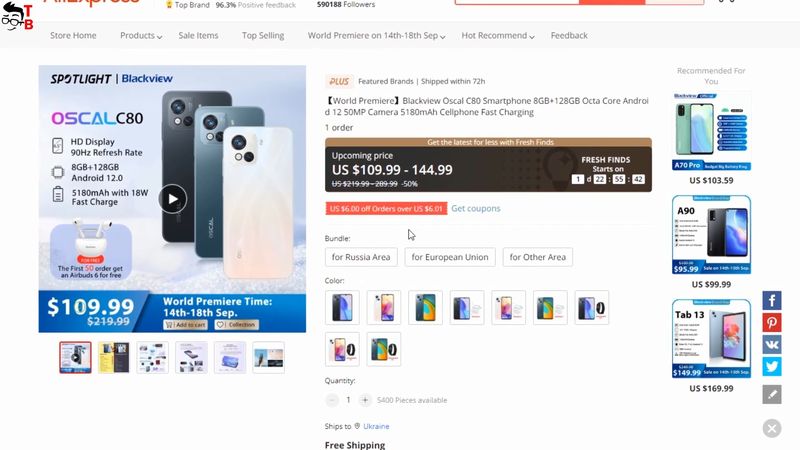This screenshot features a comprehensive view of an online store's promotional page. In the upper left corner, there is an illustration of a smiling boy with black hair and glasses. To the right of this illustration, the text reads "Top Brand 96.3% positive feedback." Below the store's header, navigation tabs include options for "Store Home," "Products," "Sale Items," "Top Selling," and "World Premiere on 14th through 18th September," followed by "Hot Recommended" and "Feedback."

On the left side of the screenshot, a promotional area highlights three cell phones displayed against a light blue backdrop. The accompanying text promotes the "Spotlight Black View Oscal C80," featuring an HD display with a 90Hz refresh rate, 6GB plus 128GB storage, and Android 12.0. The price is prominently displayed at $109.99 on a blue banner beneath the cell phones. 

Adjacent to the promotional section, additional text encourages customers to "Get the Latest for Less with Fresh Finds," reinforcing the store's commitment to offering up-to-date and budget-friendly products. The upcoming "World Premiere" event is also highlighted from the 14th through the 18th of September, emphasizing a limited-time opportunity for shoppers.